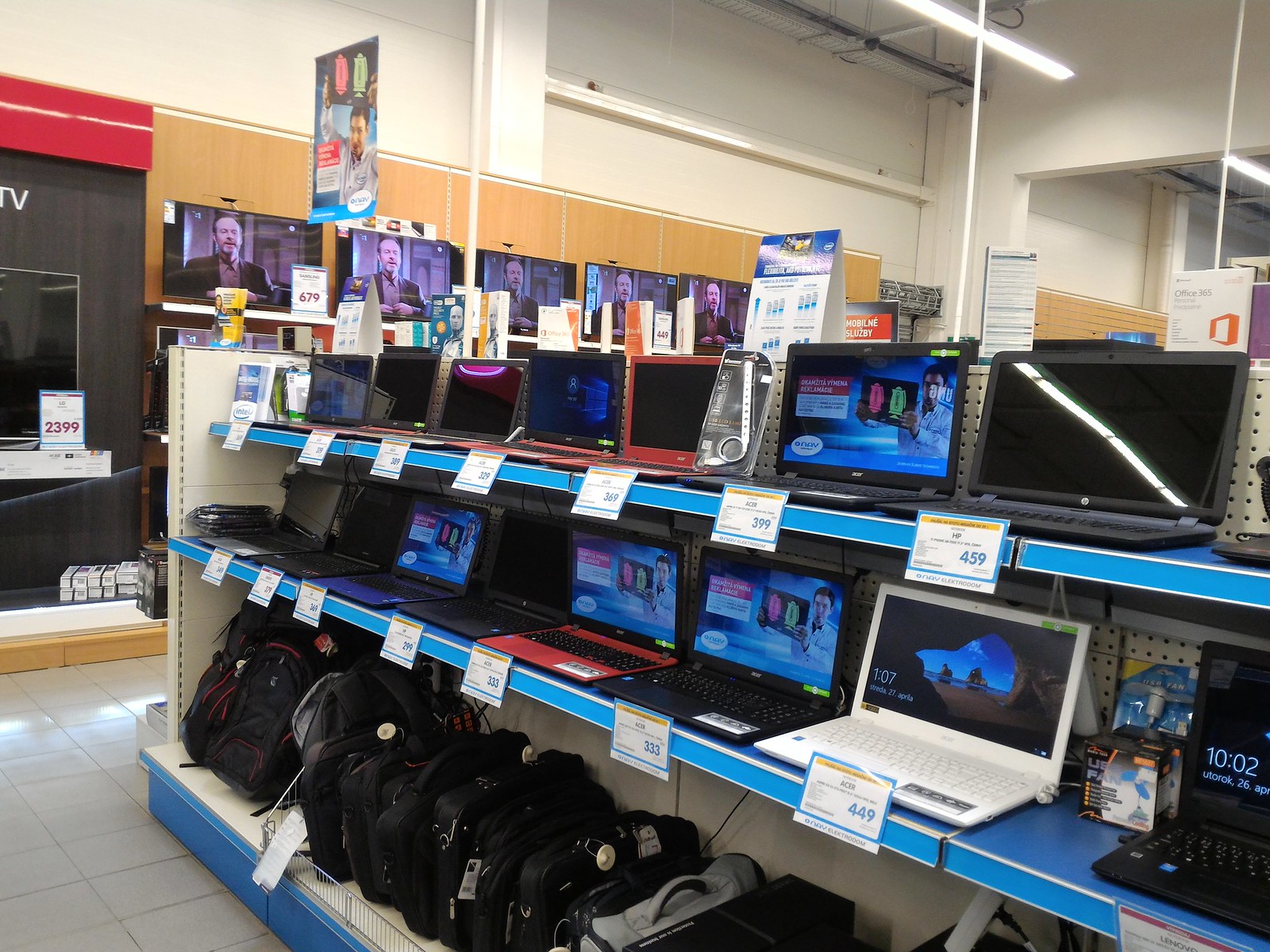Inside a large electronics store, a well-lit, detailed scene reveals rows of organized merchandise. The store has white ceilings with fluorescent lights and predominantly white upper walls, though a section features some red accents. In the background, a series of TVs are mounted against a brown wall. These TVs display the image of the same person in a suit, appearing at least five times, and one shows a price tag of $2399.

The foreground is dominated by three diagonal shelves extending from the lower right towards the upper left corner. The top shelf holds around ten laptops, mostly black except for one red model. Price tags are visible, ranging from $398 to $459. The middle shelf also displays laptops, including a distinct white one, with prices such as $239, $333, and $449. One laptop's screen indicates the time as 10:02. 

The bottom shelf features a collection of black and gray laptop bags and backpacks. The store's floor consists of white and gray tiles, clearly visible in the lower left corner of the image.